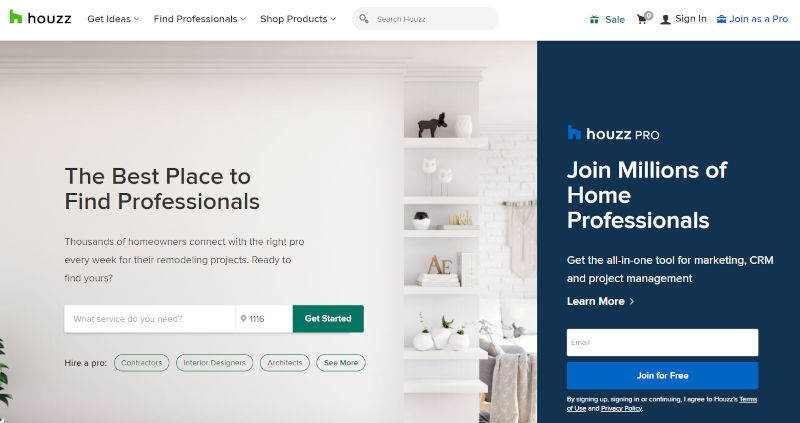The screenshot from the Houzz website captures the homepage's user interface. In the upper left-hand corner, the Houzz logo is prominently displayed next to the company name, "Houzz." A row of navigational tabs is located at the top of the page, including options like 'Get Ideas,' 'Find Professionals,' and 'Shop Products.' Adjacent to these, a search bar allows users to 'Search Houzz.'

In the upper right-hand corner, several buttons are available: 'Sale,' a shopping cart icon, 'Sign In,' and 'Join as a Pro.' 

Below this header section, the left side of the page features a photo of a modern wall with stylish shelves. Overlaid text states, "The Best Place to Find Professionals," highlighting that thousands of homeowners utilize the platform weekly for their remodeling projects. Beneath this text, there is a text box titled 'What Service Do You Need?' where users can input relevant details, followed by a field to enter a zip code and a 'Get Started' button.

On the right side of this section, a promotional message for 'Houzz Pro' invites professionals to join millions of home service experts on the platform. It highlights the all-in-one tool for marketing, CRM, and project management. This segment includes a 'Learn More' button, a text box for entering an email address, and a 'Join for Free' button.